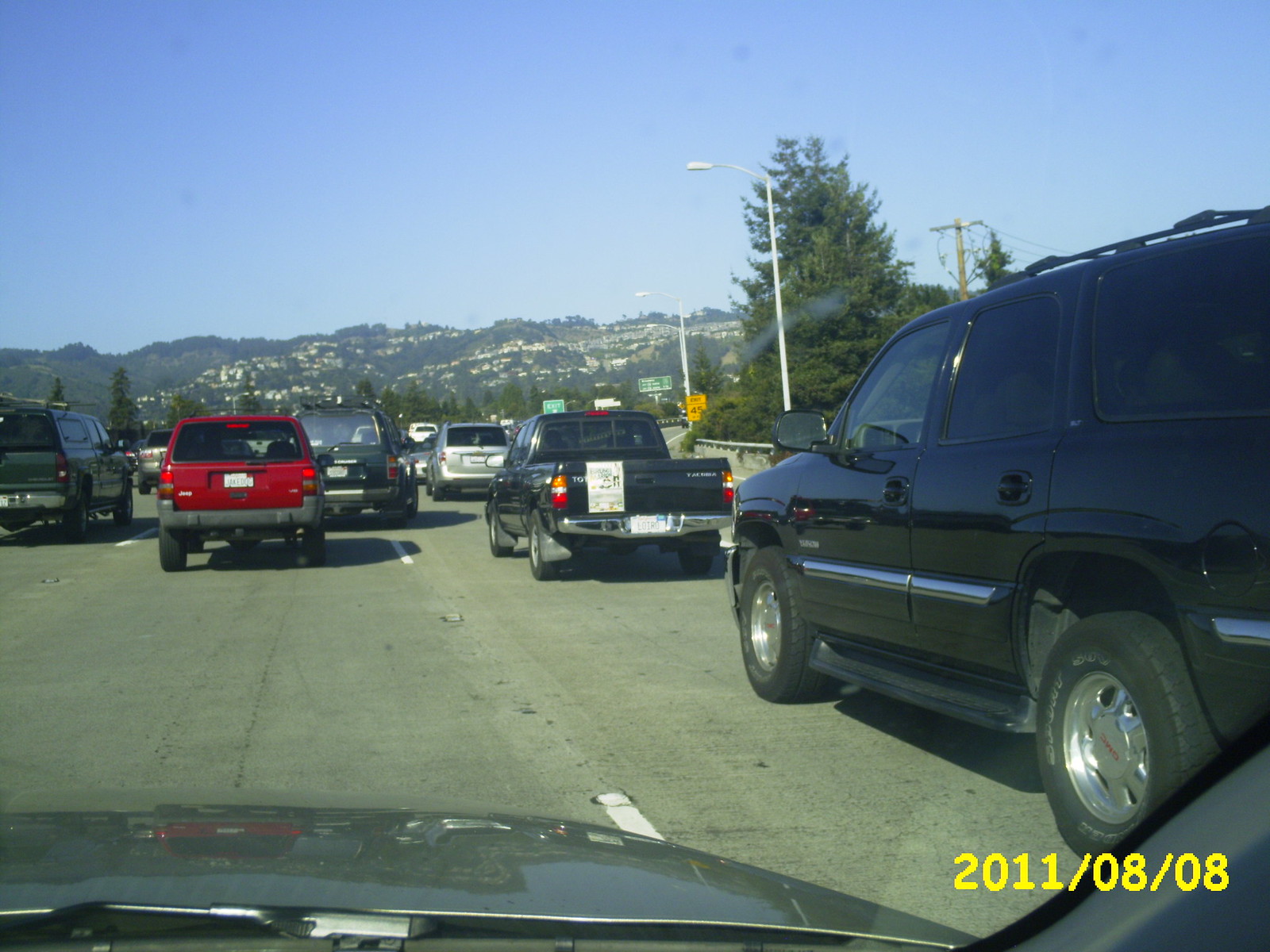Captured on a car's dash cam on August 8, 2011, this image portrays a congested interstate scene. In the bottom right corner, the date stamp confirms the timeframe. The car is caught in a traffic jam, flanked by various vehicles. To the right of the camera, a black SUV is visible, with a black pickup truck sporting a white sign on its back ahead of it. Directly in front of the camera is a red SUV, likely a Jeep, and to its left is another pickup truck, this one equipped with a bed cover. The traffic extends endlessly into the distance, suggesting all vehicles are at a standstill. The backdrop features a clear, blue, cloudless sky and some distant mountains. On the far right side of the image, a solitary tree and several street lights line the edge of the interstate, adding context to the location and surroundings.